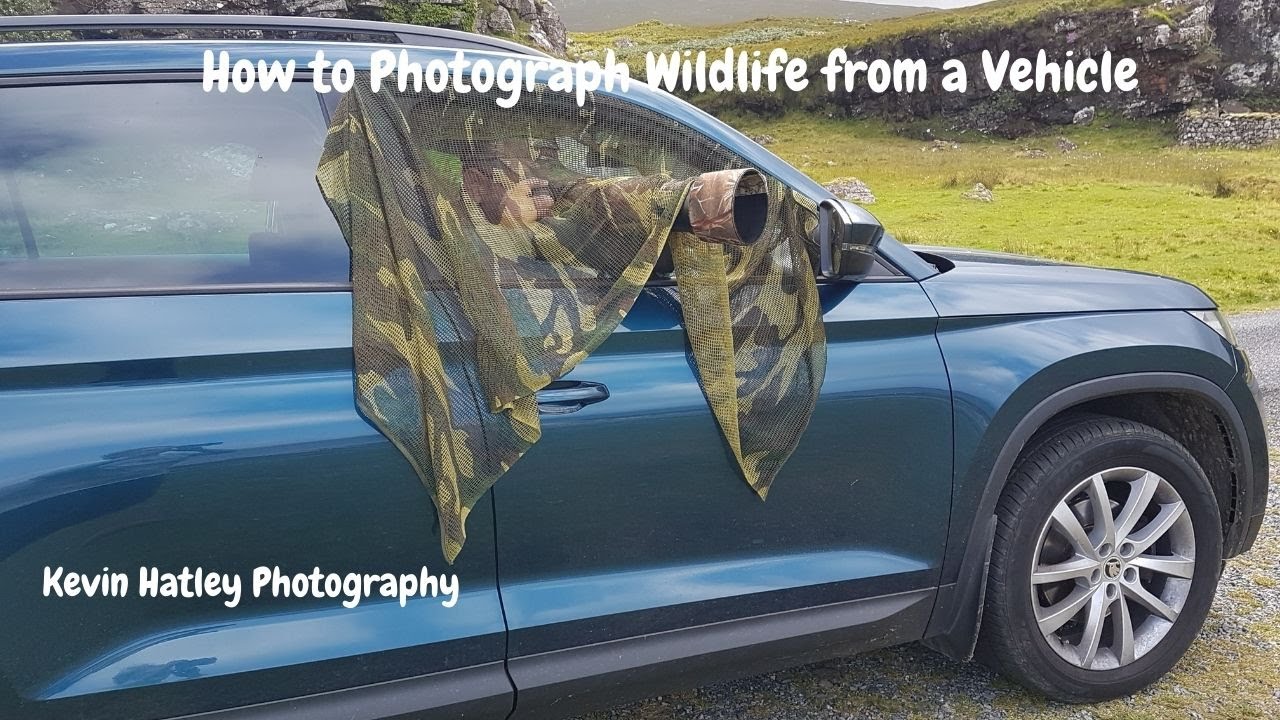The image captures a dark blue SUV parked on the side of what appears to be a street bordered by a curb. The vehicle is situated on light green-tan grass, with additional greenery and rock formations visible on the right and left sides. Through the passenger window, a photographer is seen holding a large camera with a significant telephoto lens, covered by a camouflage net to possibly shield from bugs. The net is thin enough to reveal the photographer's silhouette, hinting at a mustache and either a hat or brown hair. The car gleams with reflections of exterior light. The photograph is overlaid with white text at the top reading, "How to Photograph Wildlife from a Vehicle," and the bottom left corner of the vehicle's back door displays the name "Kevin Hatley, Photographer" in white font. The background includes a lawn leading up to a hill with stone edges, adding a natural setting to the scene.